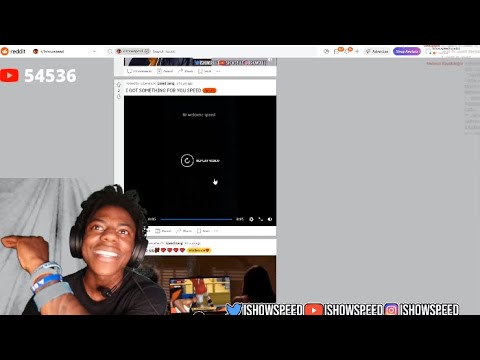A screenshot from a multi-platform social media dashboard showing a content creator's profiles on various networks. The interface backdrop is primarily white, featuring several circular and oval icons. In the top left corner, there's a red icon alongside a gray oval and a purple graphic. Central to the image are stats for YouTube, indicating a subscriber count of either 100,004 or 54,500. Gray-edged text fields denote the user's presence on different platforms. At the bottom left, a label resembling a gray blanket reads “Twitter.” 

The lower section of the screenshot includes a person wearing headphones and a black shirt, adorned with multiple wristbands, presumably the content creator. Beside this person’s image, there are recurring tags across each platform: “IShowSpeed” for YouTube, Twitter, and Instagram. Additionally, there’s a subtle, squiggly animation, possibly signifying activity or content syncing across these platforms.